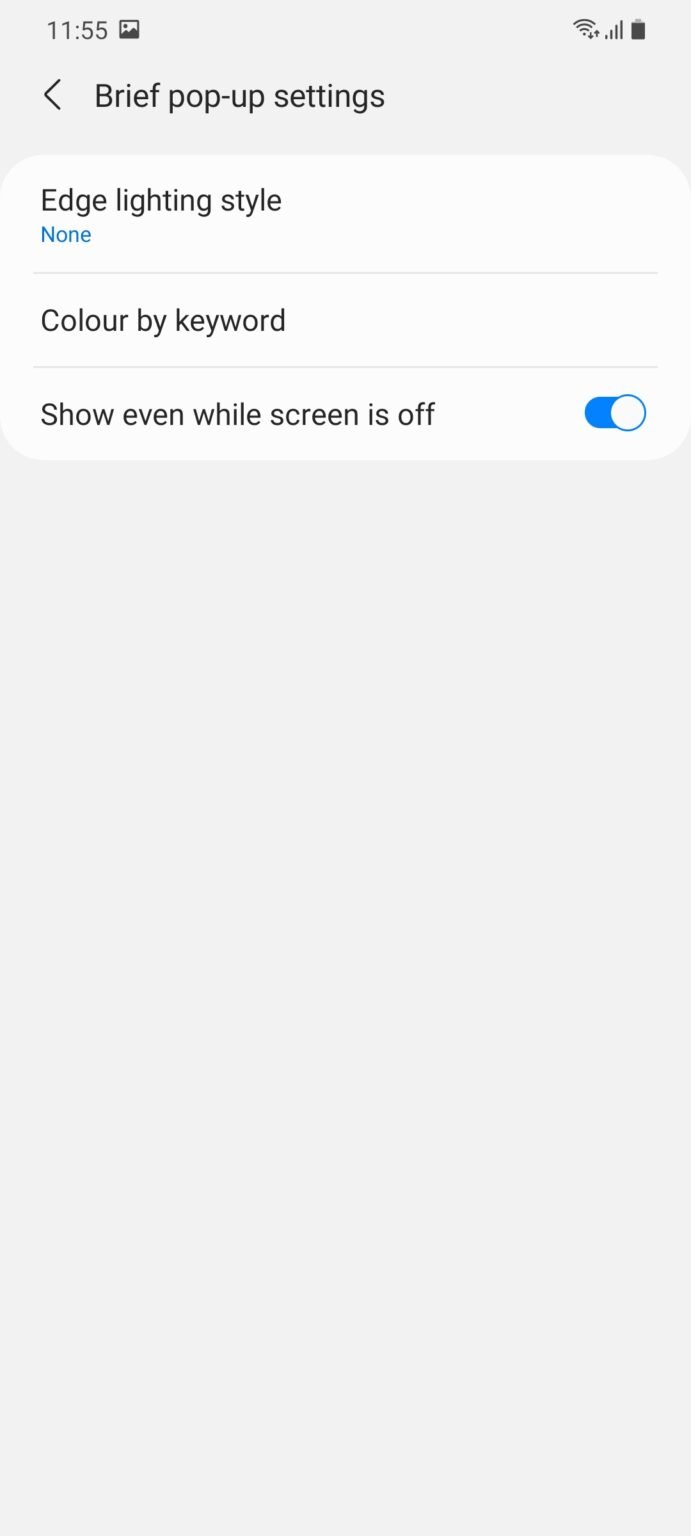In this photo, we see a detailed screenshot of a cell phone's screen. The image focuses solely on the screen's contents, excluding the physical attributes of the phone itself, but includes typical cell phone status icons. 

In the upper-right corner, displayed in black font, the time reads 11:55. Adjacent to the time is a small black screenshot icon. Moving further to the right, the cell phone reception icon shows four bars, indicating a strong signal. Next is the Wi-Fi icon, which also displays full bars, accompanied by small up and down arrows suggesting data transfer activity.

In the upper-left corner, the battery icon is visible. Beneath the status bar, in black font, appears a brief pop-up settings menu with an arrow pointing to the left, indicating a back option. The menu consists of three sections. 

The first section is titled "Edge lighting style," which is set to "Color by keyword." Below that, there is an option labeled "Show even while screen is off" with a corresponding toggle switch, which is currently turned on, indicated by a checked mark.